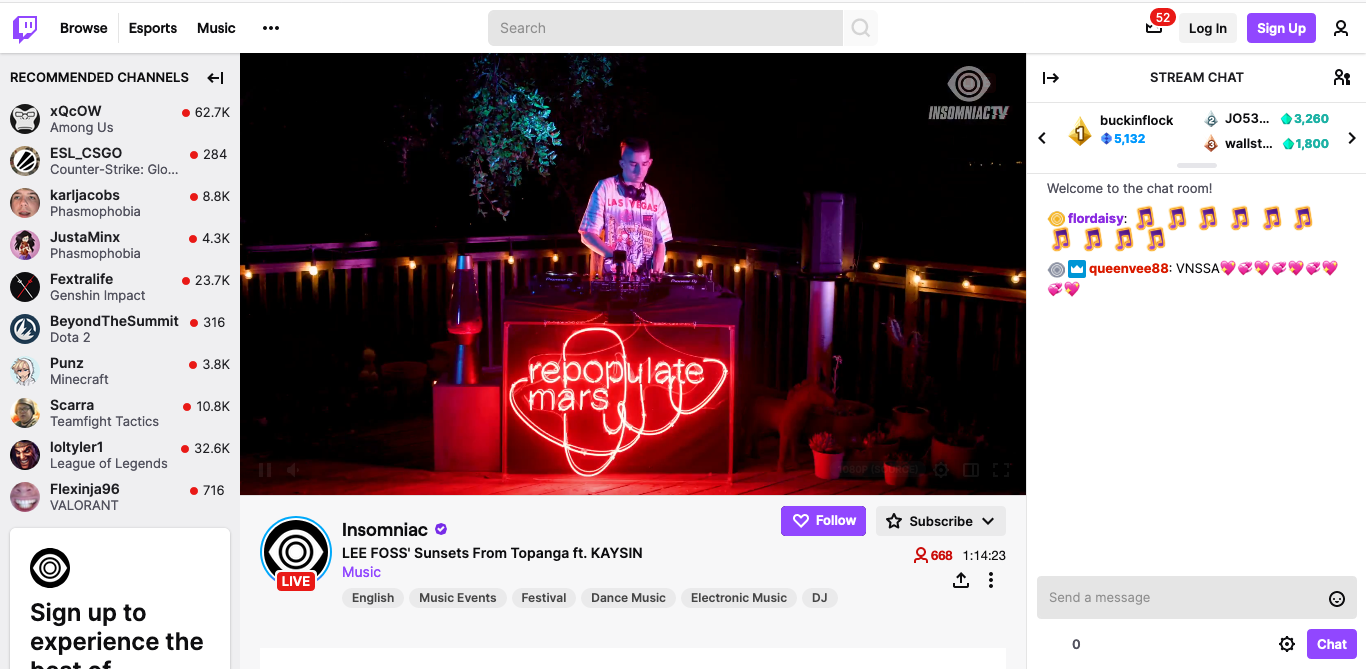This image depicts a vibrant and feature-rich webpage on Twitch with a primarily white background, dotted with gray boxes. At the top of the page, there are prominent sections labeled "Browse," "Esports," and "Music," catering to varying user interests. A conspicuous search box sits ready to help users explore content.

In the upper right corner, a notification button displays the number "52," indicating numerous updates or messages, alongside login and signup options.

The focal point of the image is an active stream chat section, where the welcome message "Welcome to the chat room!" leads comments from users such as FloraDaisy, who has shared music emojis, and Queen V88, who has enthusiastically posted "Vinsa" accompanied by an array of pink heart emojis. Below these interactions, a text box invites users to send their messages.

The main content of the stream reveals the channel titled "Insomniac," currently showcasing "Lee Foss Sunsets from Topanga featuring Kaizen." This stream is affiliated with tags like "English," "Music Events," "Festival," "Dance Music," "Electronic Music," and "DJ," which helps users navigate to similar content.

Adjacent to the chat, a "Recommended Channels" section lists various channel names along with their subscriber counts, offering users personalized viewing suggestions.

A partially visible box prompts users to "Sign up to experience," hinting at more features only available to registered users. Dominating the visual field of the stream is an image showing a large crowd and a DJ booth emblazoned with a red sign declaring "Repopulate Mars," adding a dynamic and exciting touch to the visual content.